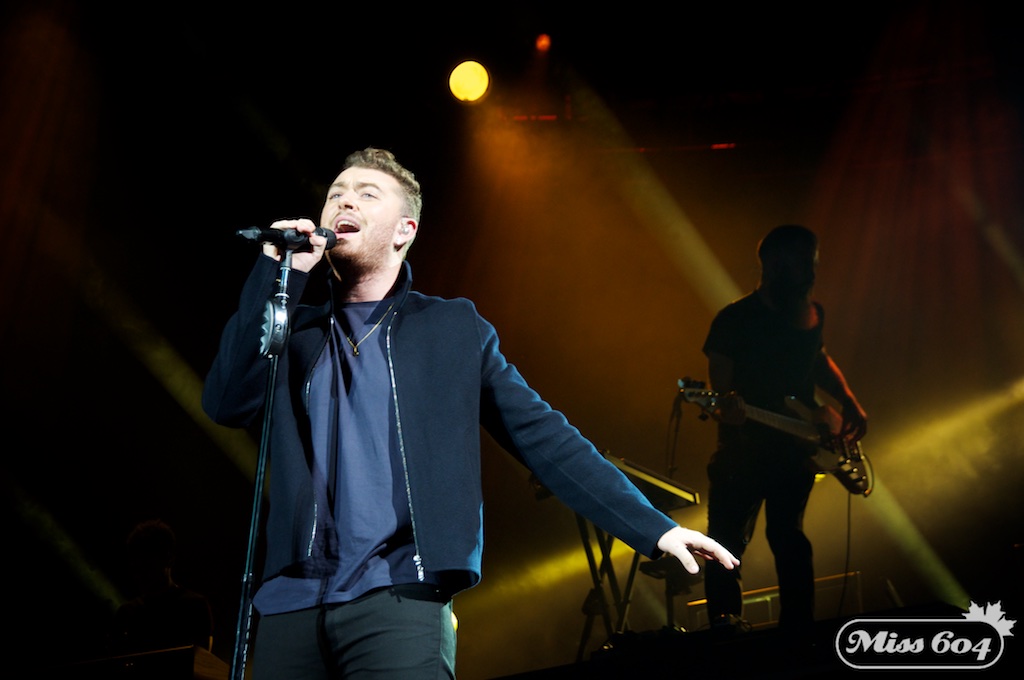A man with a mustache and a slight beard is performing on stage, illuminated under the spotlights. His light brown hair is shaved short on the sides and spiked on top. He wears black pants, a navy blue t-shirt, and a darker navy sweatshirt jacket with a silver zipper. A gold necklace hangs around his neck. Gripping a microphone on a stand, he sings passionately. Behind him, on the right side, a guitarist or bassist stands in silhouette, adding depth to the dimly lit background, where yellow spotlights create cross beams. A keyboard is also visible on stage. The photograph is marked with a logo in the bottom right corner reading "Miss 604."